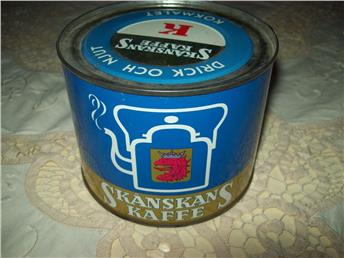In this detailed image, a metal canister of coffee takes center stage. The canister is predominantly blue, with a gold strip encircling its base. At the top, the blue surface features white lettering in a foreign language, stating something akin to "Drik Oost Noekt." The focal point of the canister’s design is a circular emblem, split into a black upper half and a white lower half, prominently displaying a red "K" at its center. 

Directly on the front, there's a detailed white outline of a kettle emitting steam, accompanied by a red illustration within a dark brown, nearly gold square. Below this illustration, an orange banner runs across the lower front, with white lettering spelling out "Skanskans Cafe K-A-F-F-E," indicating the product's name. The canister rests on a light brown surface with a circular, stone-like pattern, reminiscent of natural stone flooring.